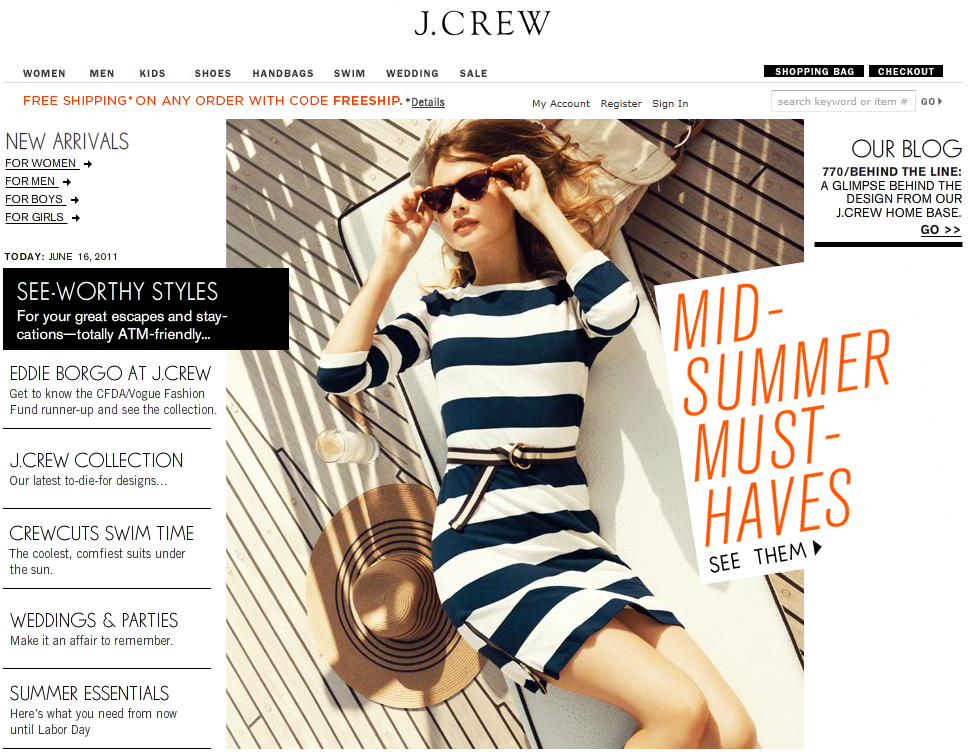On the J.Crew website, the header prominently features the J.Crew logo in black font on a white background. Below the logo, there is a sleek navigation menu with options for Women, Men, Kids, Shoes, Handbags, Swim, Wedding, and Sale, all in black text. To the far right of this menu, two black buttons labeled "Shopping Bag" and "Checkout" are situated.

Beneath the navigation menu, a red banner announces, "Free shipping on any order with code FREESHIP," accompanied by a "Details" link on the right. Adjacent to this banner are additional menu options: My Account, Register, and Sign In.

The majority of the page is dominated by a central photograph of a woman reclining on what appears to be a deck. She has blonde hair, wears sunglasses, a white and blue dress, and a hat rests beside her. To the right of this image, text reads, "Midsummer Must-Haves," along with a "See That" link.

To the right of the photograph, there is a section titled "Our Blog" with some brief information. On the left side, a pane labeled "New Arrivals" is positioned, listing clickable links for Women, Men, Boys, and Girls.

Further down the page, a black box with white font highlights "Seaworthy styles for your great escapes and staycations. Totally ATM friendly." Below this section, visitors can explore five different categories: Eddie Bargo at J.Crew, J.Crew Collection, Crewcuts, Swim Time, Weddings and Parties, and Summer Essentials.